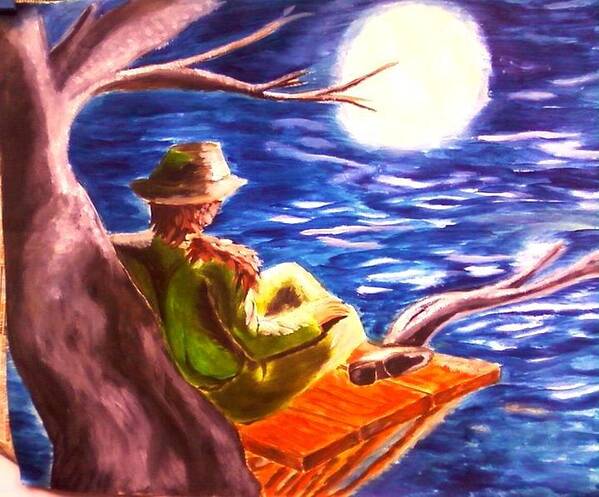The painting, likely an acrylic work, depicts a solitary figure sitting cross-legged on a bright orange wooden platform built on one of the bare, muddy auburn-colored branches of a tree. The tree, devoid of leaves, extends its branches into the night sky where a luminous full moon casts its light. The figure, donned in greenish-yellow attire with orange shading on the hat and back of the jacket, appears to have a furry visage, suggesting a transformation or a mystical element. The figure gazes thoughtfully at the moon which reflects on the blue and purple waters below, adding a serene and ethereal quality to the scene. The clear brush strokes contribute to the painting's rich texture and vivid detailing.